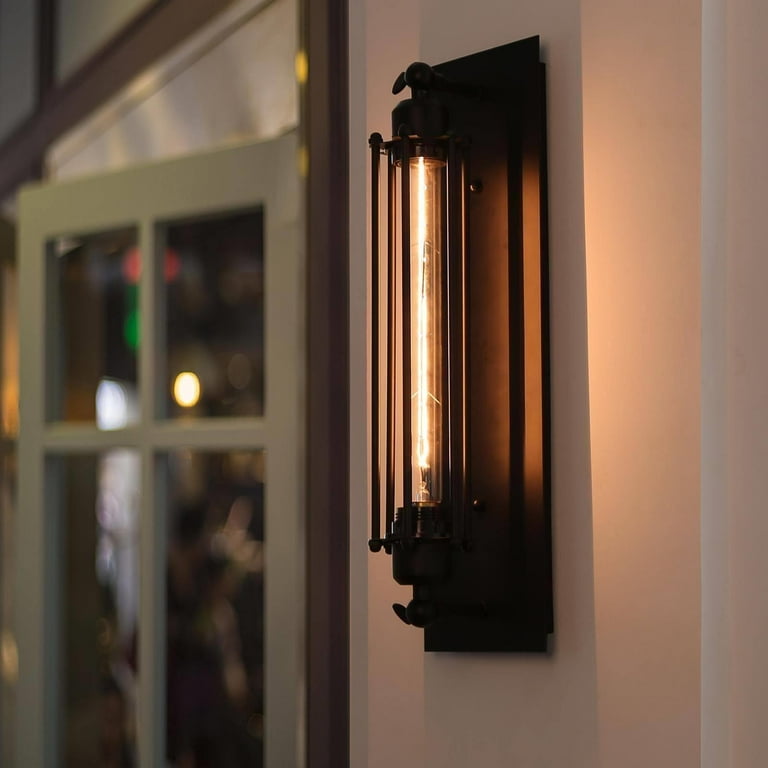This color photo, captured outdoors, displays a prominent, bright light fixture on a white or beige wall, suggesting it could be part of a house, a restaurant, or a bar. The central focus is a tall, rectangular, metal sconce featuring a thin, long tube light at its center. The light, possibly a neon or arc lamp characterized by an electric arc between electrodes, shines brightly. Notably, there is a green door with four glass panels on the left side of the frame, slightly out of focus, adding context to the setting. The fixture stands out for its elegant design, unusual for a typical residence, thus hinting at a commercial or hospitality setting.